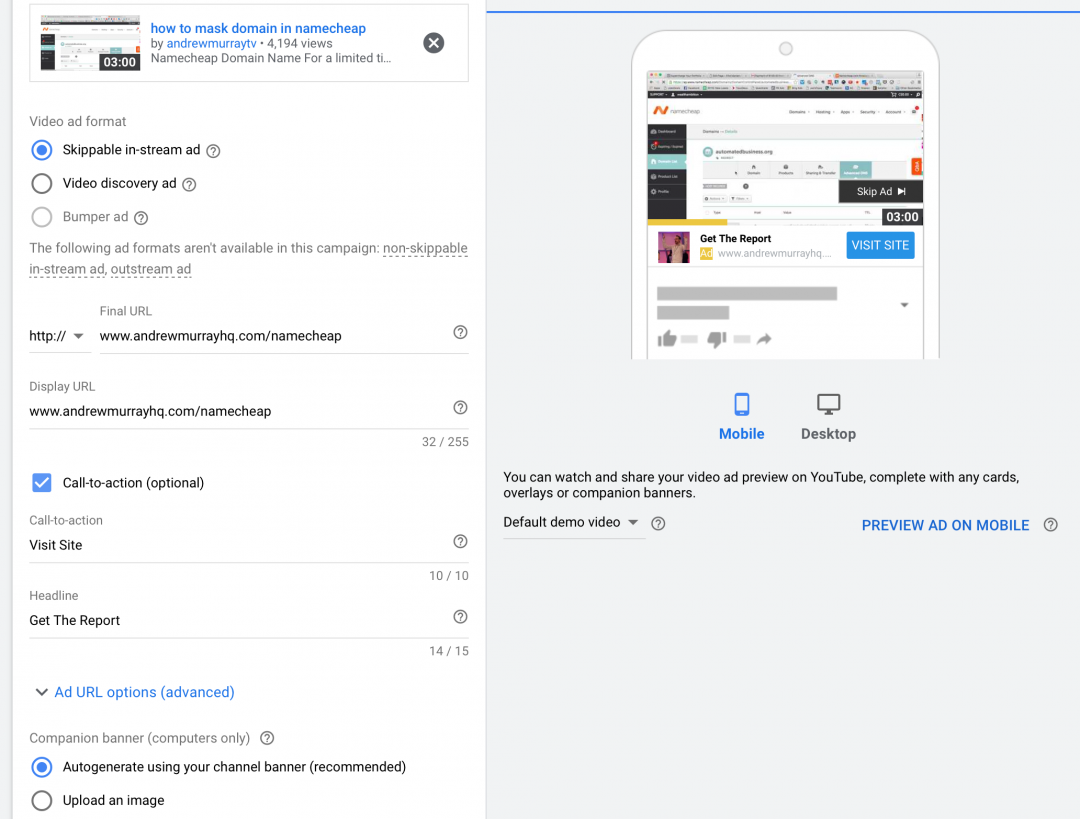A detailed screenshot of a video advertisement creation program is presented, primarily featuring a user interface with a clean white and light gray aesthetic, complemented by black text and various blue hyperlinks. In the top left corner, a small embedded video, similar to a YouTube format, is visible. The video is titled "How to Mask Domain in Namecheap" by Andrew Murray TV and has garnered 4,194 views. Below this, the selected video ad format is a “Skippable In-stream Ad,” with options for “Video Discovery Ad” and “Bumper Ad” also available through radio buttons. Notably, certain ad formats like “Non-skippable In-stream Ad” and “Out-stream Ad” are marked as unavailable for the current campaign.

Adjacent fields are provided for inputting the Final URL and Display URL, pointing to the target destination of the ad. A checkbox labeled “Call to Action” is checked, indicating this is optional; it contains fields defining the call-to-action text “Visit Site” and the headline “Get the Report.” Additional options include “Add URL Options (Advanced)”, an option specifically for “Companion Banner (Computers Only)” with the selected choice “Auto-generate using your channel banner (recommended)” standing out, and an “Upload an Image” button.

On the right side, a preview image displays a mobile device showcasing how the ad would appear on YouTube, complete with toggles to view the preview on either mobile or desktop. It highlights the ad’s ability to appear complete with any cards, overlays, or companion banners added. Below this, additional buttons are available, including an option for the “Default demo video” and a “Preview Ad on Mobile” button, allowing further interactive exploration of the ad’s presentation.